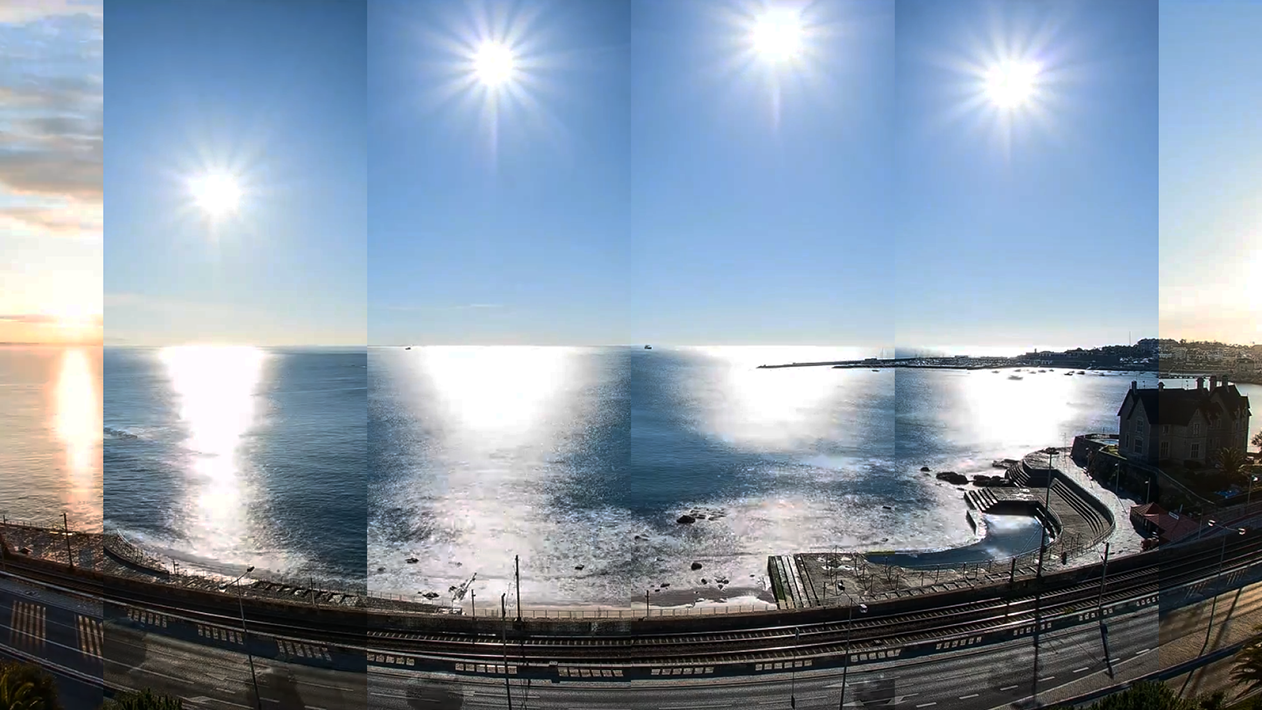The image is a horizontally rectangular photograph depicting a lakeshore scene that has been visually manipulated by superimposing twelve distinct, rectangular segments. These segments appear to show different stages of a sunrise and sunset, creating a collage-like effect. The photograph captures an industrialized lakeshore with a concrete road, busy with cars traveling in both directions. Toward the left, a peninsula extends into the lake, with a building prominently positioned in the foreground. The segmented photos at the top of the image sequentially illustrate various positions of the sun, ranging from its ascent in the morning to its peak at noon, and then its descent into evening. The sun is depicted as a bright white orb, transitioning to shades of orange at the horizon during its initial rise and final set. This creative artwork melds together the changing light and times of the day into a cohesive, yet fragmented portrayal of a bustling lakeshore environment.